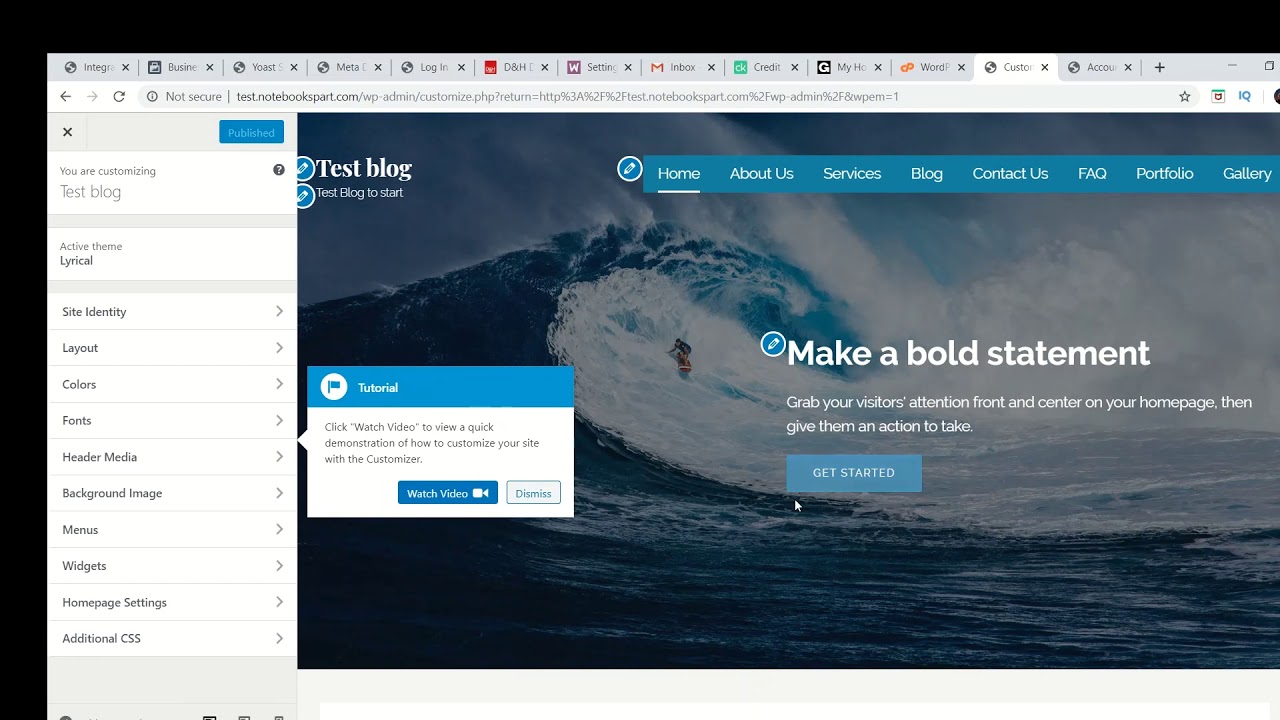This image is a screenshot of a webpage displayed on a laptop. The photo itself features a black background on the left and top edges and fades to an undefined background at the bottom. At the top of the screen, a gray bar contains approximately twelve open tabs.

The left side of the webpage showcases a vertical sidebar with a gray border encompassing several white boxes. At the top right of this sidebar, a blue button with white text appears, which seems to say "Published," although the text is somewhat blurred. Just below, a white bubble reads "You are customizing" with "Test Blog" beneath it. Following that is another white bubble indicating "Active themes," specifying the theme as "Lyrical."

The sidebar continues to present various customization options including "Site Identity," "Layout," "Colors," "Fonts," "Header," "Background," "Menus," "Widgets," "Homepage Settings," and "Additional CSS," each accompanied by arrow icons for further details.

In the main content area of the page, the title "Test Blog" is displayed above an image of a person surfing a giant wave, which is presented in landscape orientation. Overlaying this image is a blue and white rectangular popup box containing a "Watch Video" icon and a "Dismiss" button.

To the right of the surfer image, white text reads "Make a bold statement," accompanied by a rectangular blue "Get Started" button with white font centered within it.